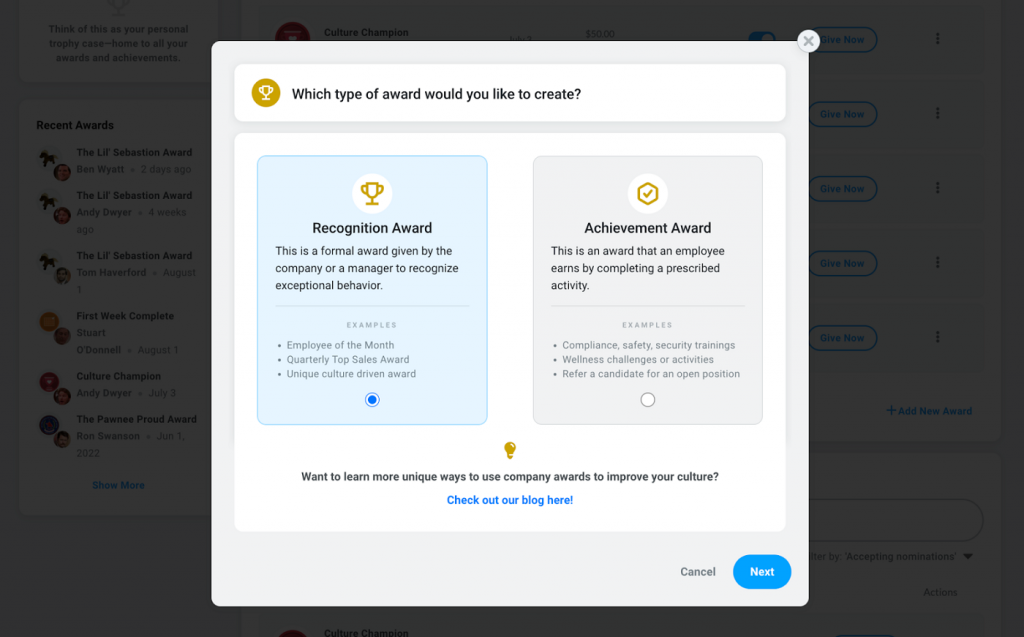The image depicts a webpage centered on the creation and selection of awards. At the top, there's a section titled "What type of award would you like to create?" Accompanying this title on the left is a small yellow emblem. 

The user is presented with two main options for types of awards: 

1. **Recognition Award**: This option is already selected and features a gold trophy emblem. The description beneath it reads, "Recognition Award: This is a formal award given by the company or a manager to recognize exceptional behavior." Examples provided include "Employee of the Month," "Quarterly Top Sales Award," and "Unique Culture-Driven Award."

2. **Achievement Award**: This option is unselected and is symbolized by an emblem with a check mark. Its description states, "This is an award that an employee earns by completing a prescribed activity." Examples include "Compliance," "Safety," "Security Trainings," "Wellness Challenges or Activities," and "Refer a Candidate for an Open Position."

At the bottom of the page, there is a section prompting users to explore more by clicking on a link to the blog, indicated by a gold light bulb icon with the text, "Want to learn more unique ways to use company awards to improve your culture? Check out our blog here."

The page also features two actionable buttons: "Cancel" and "Next," the latter highlighted in bright blue with white text, positioned at the bottom-right corner of the screen.